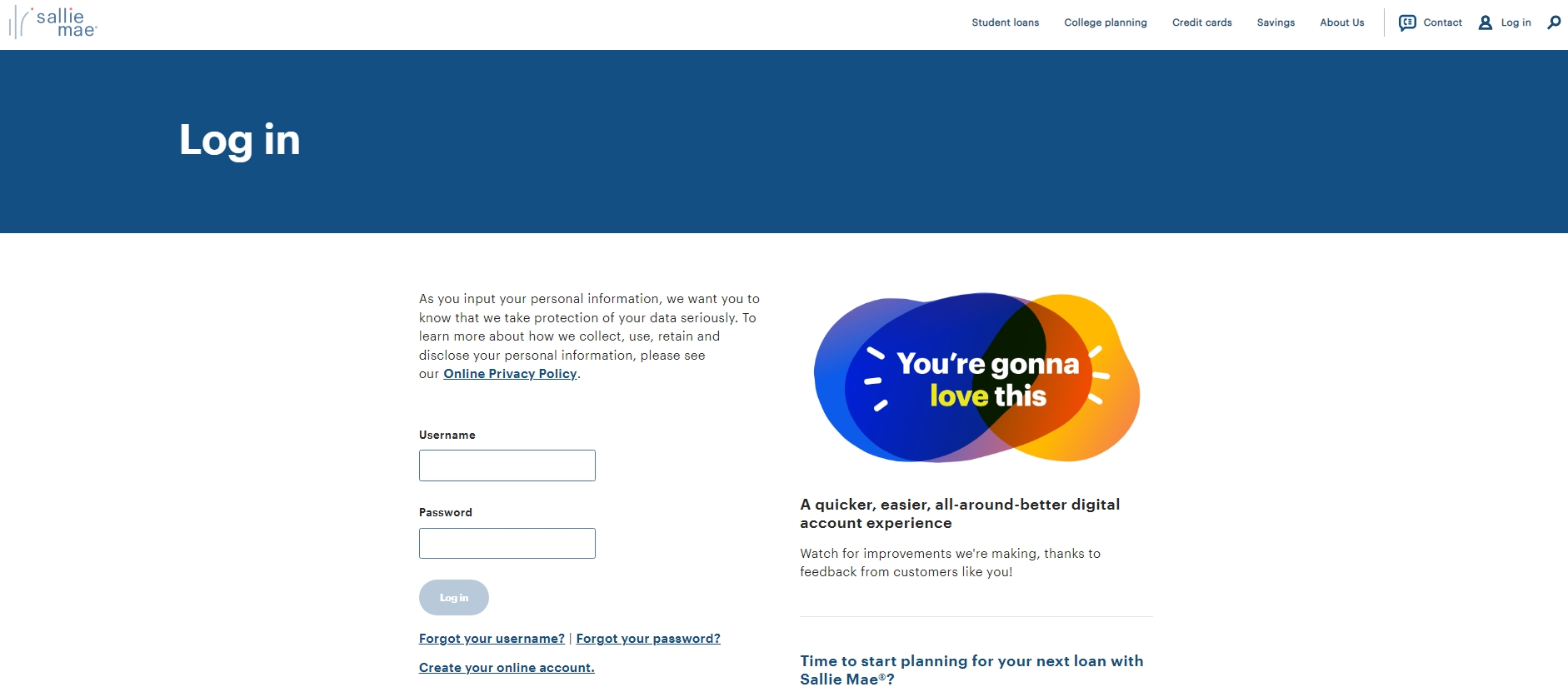This is a detailed description of a screenshot taken from a laptop showing the Sallie Mae website. 

In the upper left-hand corner, there are two straight lines followed by a curved line with a red dot above it. The website header displays the name "Sallie Mae" written in lowercase letters ('sallie mae'), in blue. To the right of the website name, there is a navigation menu with several options: "Student Loans," "College Planning," "Credit Cards," "Savings," "About Us," "Contact," and "Login," followed by a search icon.

Prominently, a large blue bar spans across the upper section of the page, containing the word "Login" in white text towards the left. Below this, the main page has a white background featuring a security notice that reads: "As you input your personal information, we want you to know that we take protection of your data seriously. To learn more about how we collect, use, retain, and disclose your personal information, please see our Online Privacy Policy," with "Online Privacy Policy" underlined and in blue.

Further down, there are login fields: one box labeled "Username" and another labeled "Password." Beneath these boxes is a light-colored oval button labeled "Login," followed by links for "Forgot your username?" and "Forgot your password?" both underlined. Additionally, there is an underlined link titled "Create your online account."

To the right of these fields, text reads: "You're going to love this," accompanied by a background of three colored blobs – light blue, purple-tinged blue, and yellow – blending into an orange hue in the middle. Below this text, there is a promotional message stating: "A quicker, easier, all-around, better digital account experience. Watch for improvements we're making thanks to feedback from customers like you. Time to start planning for your next loan with Sallie Mae?" with the question mark in blue.